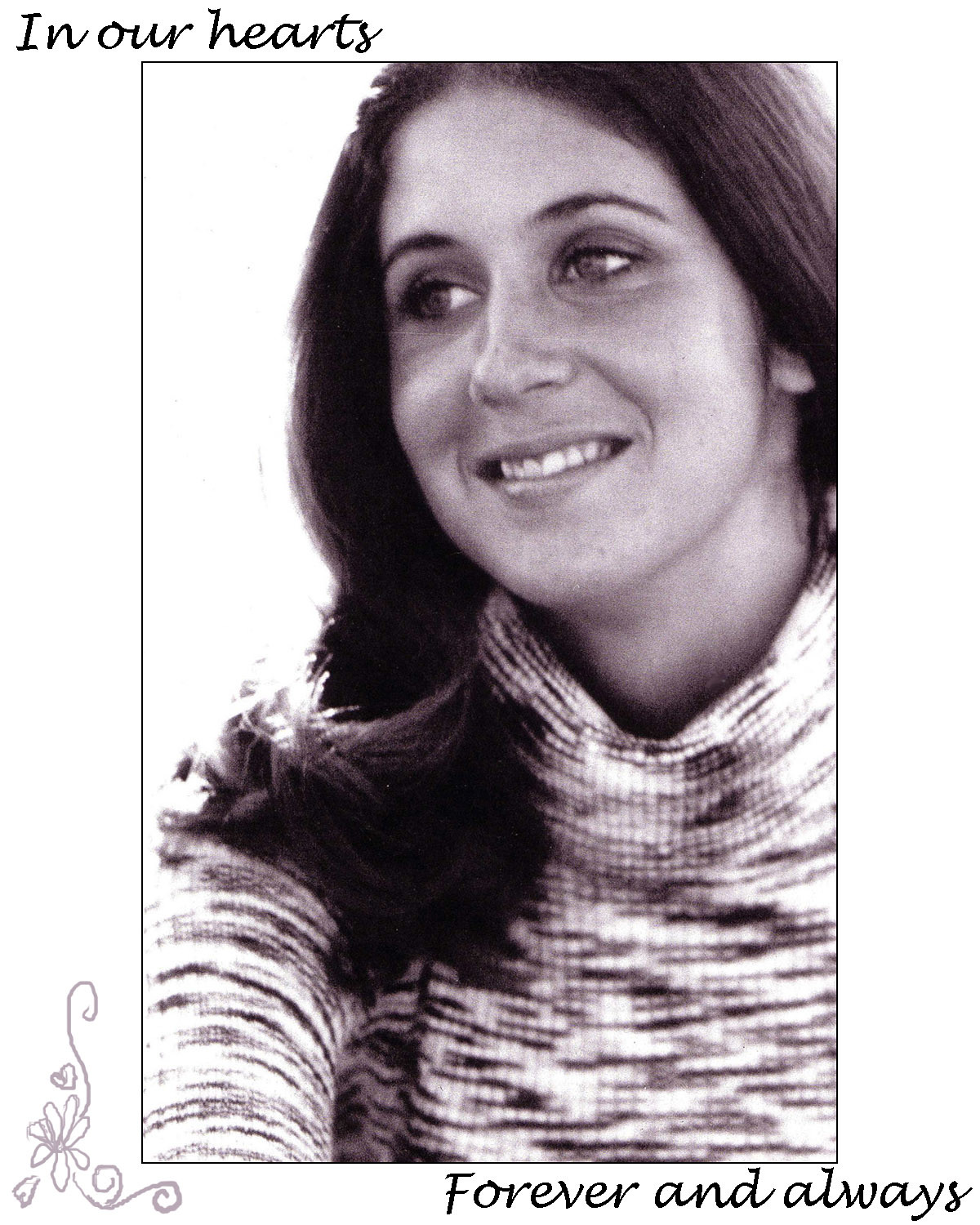This black-and-white photograph features a woman, likely from the 1970s, judging by her hairstyle and clothing. The image is bordered by a black outline and centered in the frame, featuring black text at the very top that reads "in our hearts" in cursive. At the bottom, the text says "forever and always." A stylized flower and some lines adorn the bottom left corner, adding subtle decorative elements.

The woman has dark, almost black hair that falls just below her shoulders. She wears a horizontally striped turtleneck sweater that has a loose fit and long sleeves. Her expression is peaceful and content, characterized by a bright, open smile that reveals white teeth. Her eyes are lively and contribute to her overall appearance of happiness and tranquility. The photo exudes a sense of ease and fond remembrance.